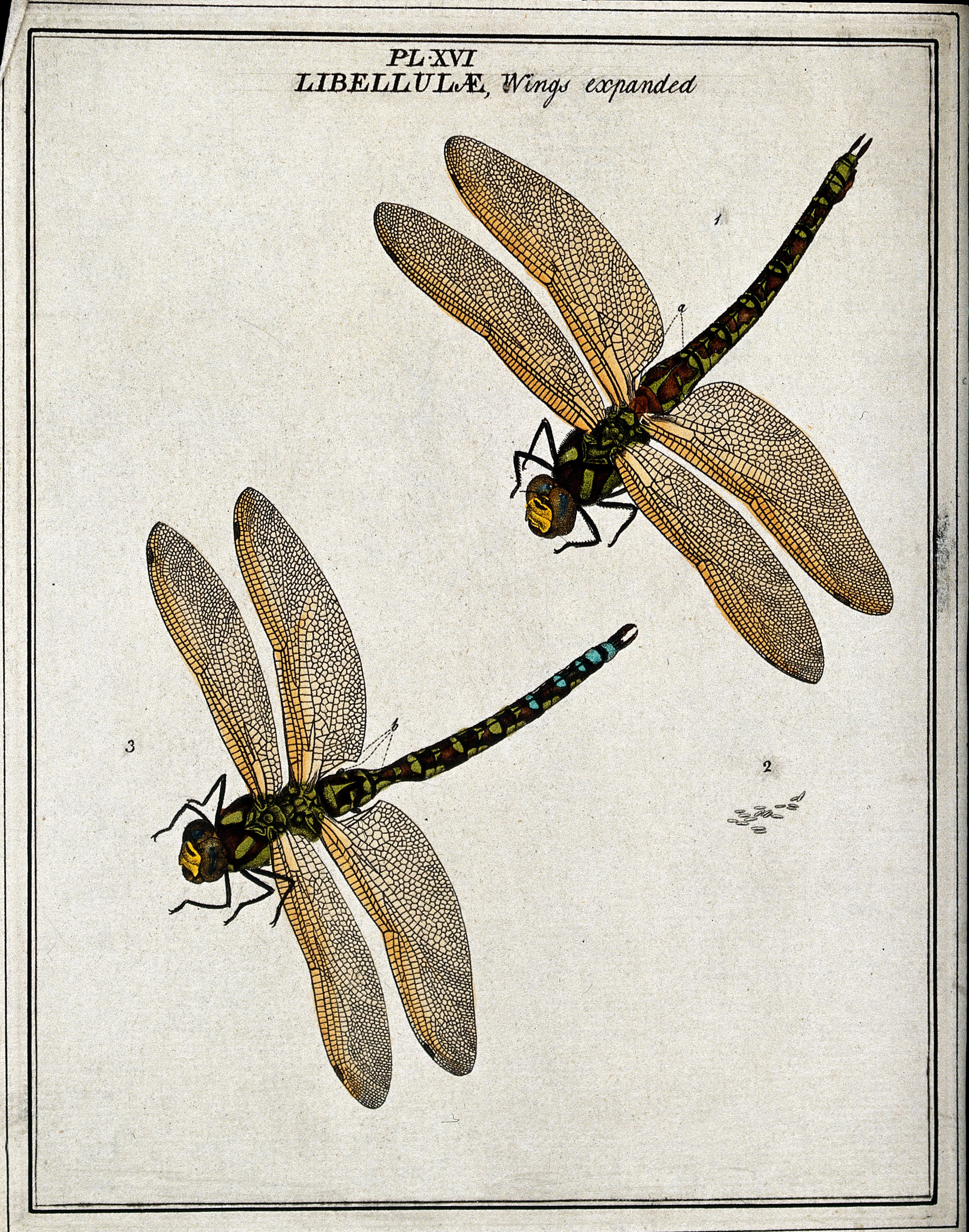This detailed caption combines the shared and specific details provided:

This antique illustration, likely sourced from an old textbook or naturalist's journal, depicts two dragonflies in intricate detail. The dragonflies, possibly rendered in a combination of painting and drawing techniques, exhibit dark green and red hues with yellow on their faces. Their segmented bodies and delicate wings are meticulously drawn, showcasing the artist's attention to naturalistic detail. The background is a grayish-tan blend, enhancing the vintage, antique feel of the image. The entire piece is framed with a black border and features text in both Latin and English; the Latin script includes "PLXVI" and "Libellium," while a prominent English label reads "Wings Expanded," likely referring to the fully extended wings of the insects. Additionally, the image is marked with numerical annotations: number 1 identifies the top dragonfly, number 3 the one below it to the left, and number 2 highlights small dotted details. The overall composition suggests the image is either part of a historical book or a poster, conveying a sense of aged elegance through its use of old golds, dark maroons, and greens.